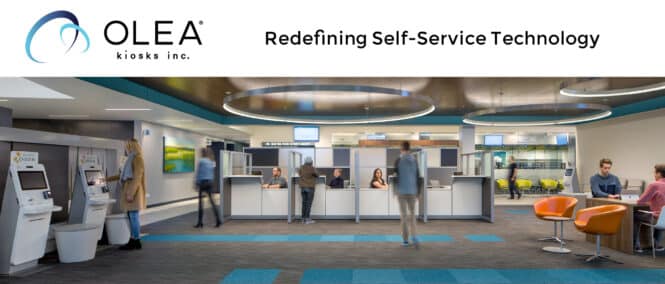The image depicts a modern, futuristic office setting, likely a reception area for a doctor's office or similar facility, equipped with advanced self-service technology. At the top left, a large, curved blue logo for OLEA Kiosks, Inc. is prominently featured, accompanied by the tagline "Redefining Self-Service Technology" in bold black letters. The scene below shows two sleek, white self-service kiosks on the left, with a woman in a tan coat, scarf, blue jeans, and black boots interacting with one of them. The carpet is gray with blue lines, and behind the kiosks, there are white partitioned desks where people are seated and others are walking around. On the right side of the image, a brown desk table with orange chairs hosts two men working on laptop computers. Overhead, circular lights illuminate the space, reinforcing the contemporary and efficient design.